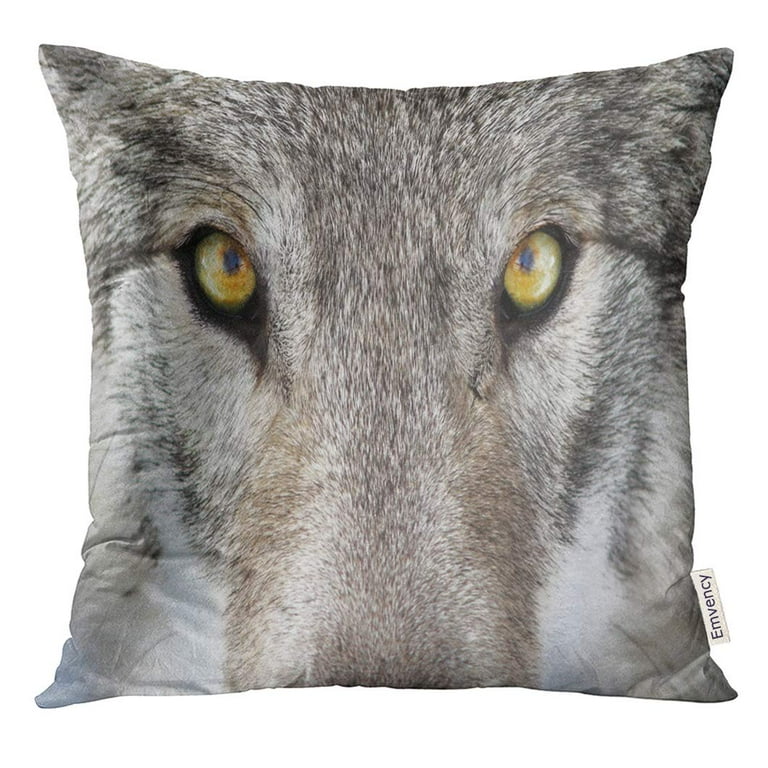This novelty throw pillow is square-shaped and portrays a striking, close-up image of a wolf's face. The wolf has a mix of gray, brown, and white fur, creating a tabby-like pattern that adds texture to the image. The eyes of the wolf, which are yellow and green with a golden hue, are the focal point, positioned towards the top of the pillow. Black rings accentuate the eyes, enhancing their glowing effect. The snout is centered but cropped off at the bottom, and you cannot see the nose, mouth, paws, or tail; only the upper face and the bridge of the snout are visible. The detailed fur patterns, including white fur on the bottom corners and varying shades of gray and brown throughout, completely fill the pillow, leaving no empty space. A small, rectangular brand tag reading "M. Vencey" in black text is attached to the bottom right corner of the pillow. The pillow is shown on a solid white background, highlighting its intricate design and making the wolf's captivating gaze stand out even more.